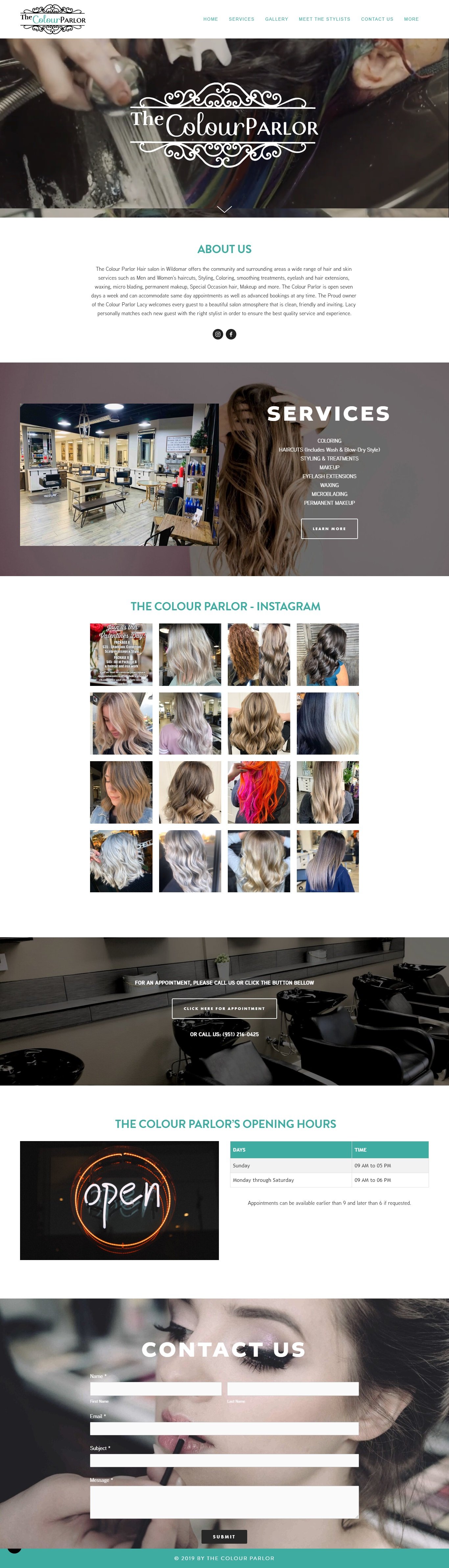Discover the Color Parlor, located in Wildomar, where “Colour” and “Parlor” are spelled the British way, adding a touch of elegance to this premier salon. This vibrant advertisement highlights the extensive range of hair and skin services offered to the community and its surrounding areas. Services include men's and women's haircuts, styling, coloring, smoothing treatments, eyelash extensions, hair extensions, waxing, microblading, permanent makeup, special occasion hair, makeup, and more.

The salon is open seven days a week, accommodating both same-day appointments and advanced bookings. Proud owner Lacey ensures a warm welcome for every guest in a beautifully maintained, clean, friendly, and inviting atmosphere. Lacey takes the time to match each new client with the perfect stylist, guaranteeing top-quality service and an exceptional experience.

The featured image showcases the spacious salon with multiple stations and hardwood flooring, emphasizing a modern and stylish environment. The Color Parlor's Instagram feed is filled with vibrant transformations, including striking hair colors such as Cruella-inspired black and white, hot pink and red, and elegant grays. One notable example features a beautiful blend of highlights and lowlights, creating a stunning and sophisticated look.

For appointments, visitors are encouraged to call or click the provided button. The salon's operating hours are Sunday from 9 a.m. to 5 p.m., and Monday through Saturday from 9 a.m. to 6 p.m. Appointments outside these hours can be arranged upon request for added convenience. An open sign prominently displayed within a distinct orange oval further invites clients to experience all that the Color Parlor has to offer. Contact information is readily available for those eager to book their next appointment.